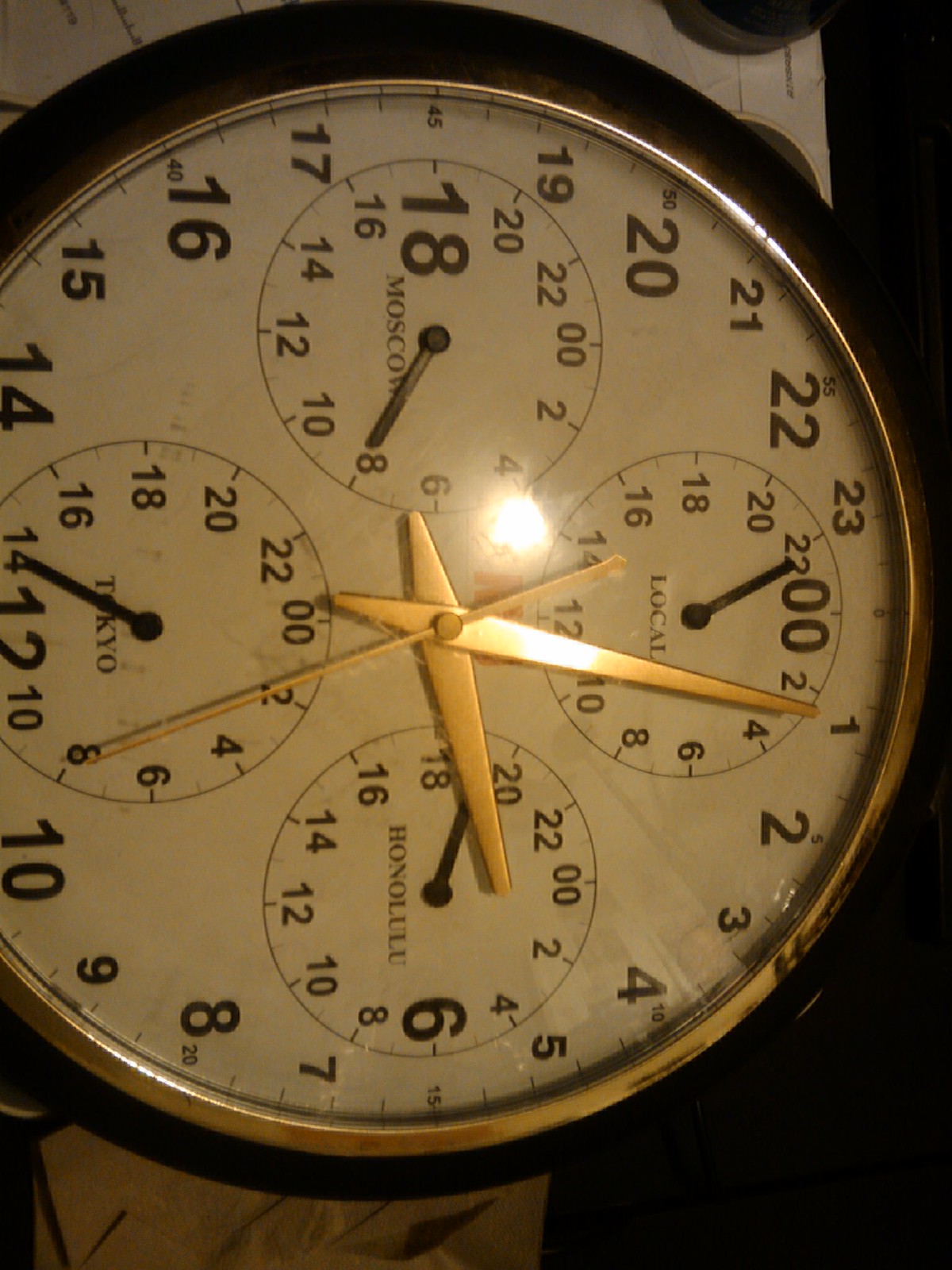This is a close-up image of an ornate clock, captured from a sideways angle. The clock itself is round and features a gold or brass rim encased in a dark wood frame, further accentuated by the same metallic finish. A clear glass cover protects the clock's face.

The clock has three gold hands indicating the hour, minute, and second, set against black numbers that uniquely range from 1 to 24. In addition to the primary timekeeping function, the clock's face is adorned with four smaller subdials, each containing its own needle. These subdials are labeled to represent different time zones: "Local" at the top, "Honolulu" on the right, "Tokyo" at the bottom, and "Moscow" on the left. This complex timepiece offers a wealth of information and showcases intricate craftsmanship.